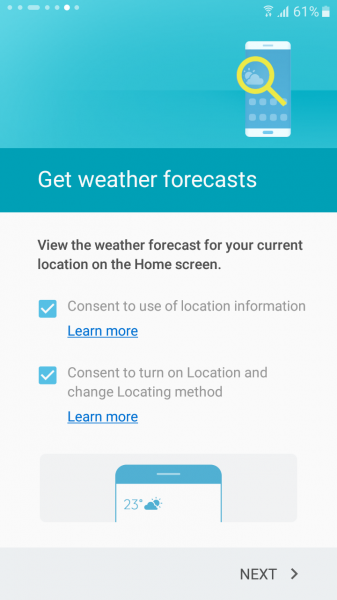The background of the image transitions through three different shades of teal, becoming lighter at the top and darker towards the bottom. On the left-hand side, there are various gray shapes: two circles, followed by an oval, two more circles, a white circle, and then another gray circle. The right-hand side features white icons for Wi-Fi signal strength and reception, displays "61%" in white, and shows a battery level that is slightly more than halfway full. At the far right, there is a phone icon with white top and bottom sections. A yellow magnifying glass is positioned over an illustration of a sun and cloud. Below this, four light blue squares are visible.

Towards the bottom of the teal gradient, the text "Get Weather Forecast" is displayed in white with a capital "G". The background then shifts to an off-white color. In black text, it says, "View the weather forecast for your current location on the Home screen." The word "View" features a capital "V," and "Home" starts with a capital "H."

Below this, there is a light blue box containing a white checkmark, and the gray text reads, "Consent to the use of location information." Underneath this text, there's a blue and underlined "Learn More" link. 

After some space, a second light blue box appears with a similar white checkmark. Beside this mark, the gray text reads, "Consent to turn on location and change locating method." Below, there is another underlined "Learn More" link in blue.

At the very bottom, there is a light gray rectangle, accompanied by a phone tab icon that is white and teal, indicating the number "23".